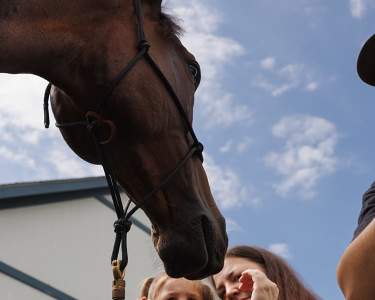The photograph is a small horizontal rectangle that features a close-up of a dark brown horse with a black bridle, leaning its head down towards two people. The horse's head is in the upper left corner, extending down towards the center of the image. To the bottom right of the horse, a little blonde girl and her mother, who has long brown hair, are gazing up at the horse. The mother's left hand is raised, as if about to pet the horse. A man's arm and the brim of his hat can be seen at the right edge of the image. The background features a light blue sky with fluffy white clouds, and a beige barn with darker wood trim partially visible in the lower left corner. The image suggests an intimate moment between the horse and the people, with vivid details enhancing the bucolic atmosphere.